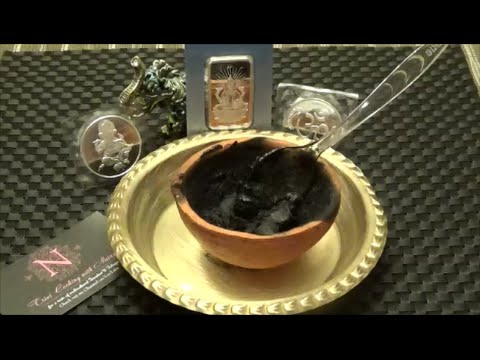The image features a striking arrangement against a black background. A gold, metal-like bowl holds a ceramic, orange-hued bowl that resembles half an orange. Inside this ceramic bowl is a black substance, possibly ink or caviar, with a clear serving spoon dipped into it, noticeably coated in the substance. Surrounding the main focus are several decorative items: on the left, a glass-encased emblem, possibly representing an angel or cherub; in the center, a silver frame containing another emblem; and on the right, a square glass item with an indistinct symbol inside. Additionally, there is a small, rectangular crystal piece with an emblem in the middle located to the right of the gold bowl. An arrangement of other statues, possibly depicting a Buddhist or Hindu deity and an elephant, adds to the eclectic display. The setup rests on a two-tone black mat with a woven appearance outlined in gold, reminiscent of a Louis Vuitton pattern. A business card with a large 'N' and illegible text lies on the mat.